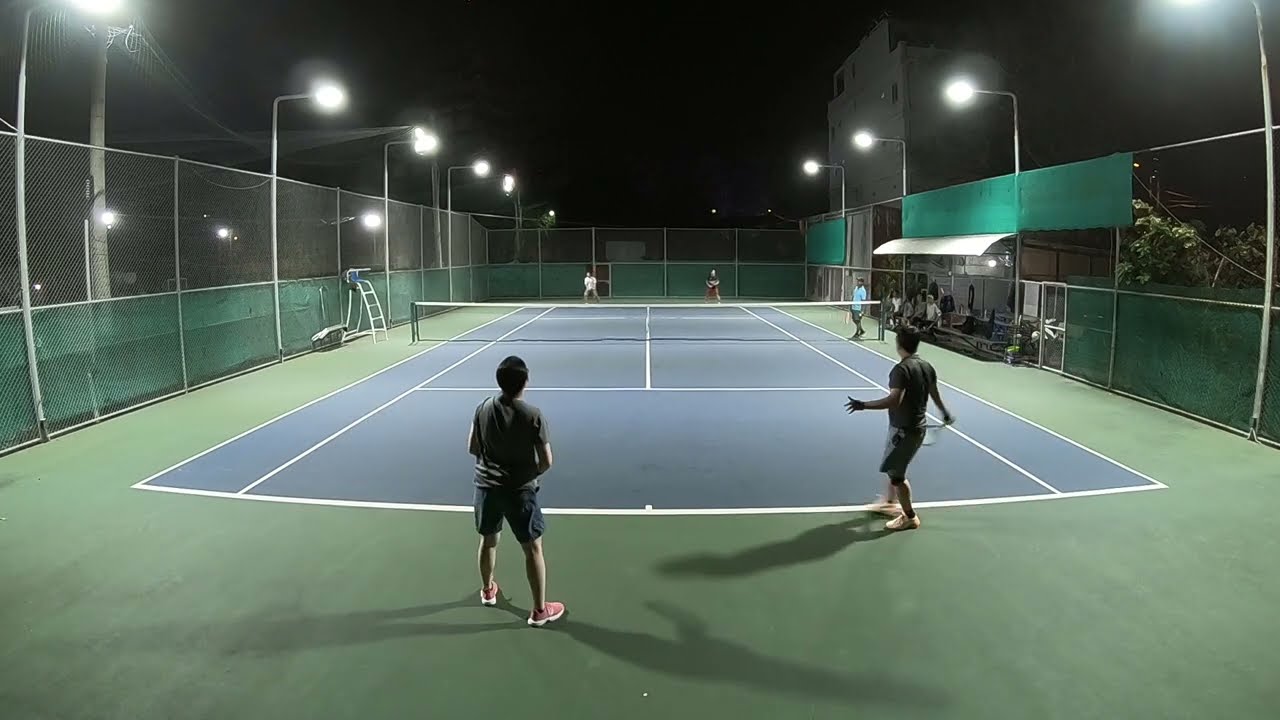The photo captures a nighttime doubles tennis match on a beautifully maintained court, characterized by its green perimeter and blue playing area. The vantage point is from one end of the court, providing a view down towards the far baseline where two players are positioned. The players in the foreground are dressed in grey shirts and blue shorts, while the opponents in the background wear a mix of white, grey, dark shirts, and dark red shorts. The court is illuminated by angled lights mounted on tall poles surrounding the area. To the left of the net stands an umpire's chair with a ladder, and on the right side, one can observe bleachers with spectators. A tall fence encircles the court, adding a sense of enclosure. In the distant background, the silhouette of a tall city building emerges against the black night sky, emphasizing the urban setting.